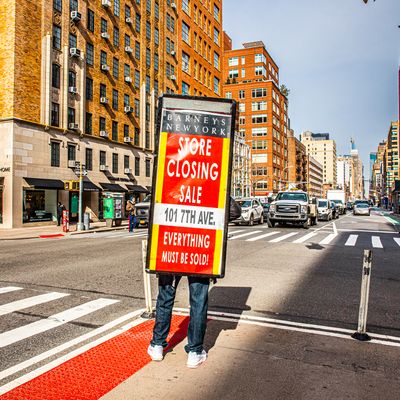In the photograph, a man stands in the middle of a busy downtown street intersection, holding a large, vertical sign advertising the "Barney's New York Store Closing Sale," located at 101 7th Avenue with the slogan “everything must be sold.” The sign is predominantly yellow and red with black and white text. The scene is set on a sunny day with a clear blue sky, casting light on the surroundings. The street is lined with rows of multi-story, orange-brick buildings featuring large shop windows and awnings on their gray cinder block ground floors. Each upper window is fitted with an air conditioning unit protruding out. In the background, a queue of cars is stopped at a traffic signal, and a fourth lane remains empty at the crosswalk where the man is standing. He is dressed in blue jeans and white sneakers. The street beneath is a concrete road with white markings, and there are electric poles, lampposts, and other street lights visible along the pavement where some cars are parked by the shops.